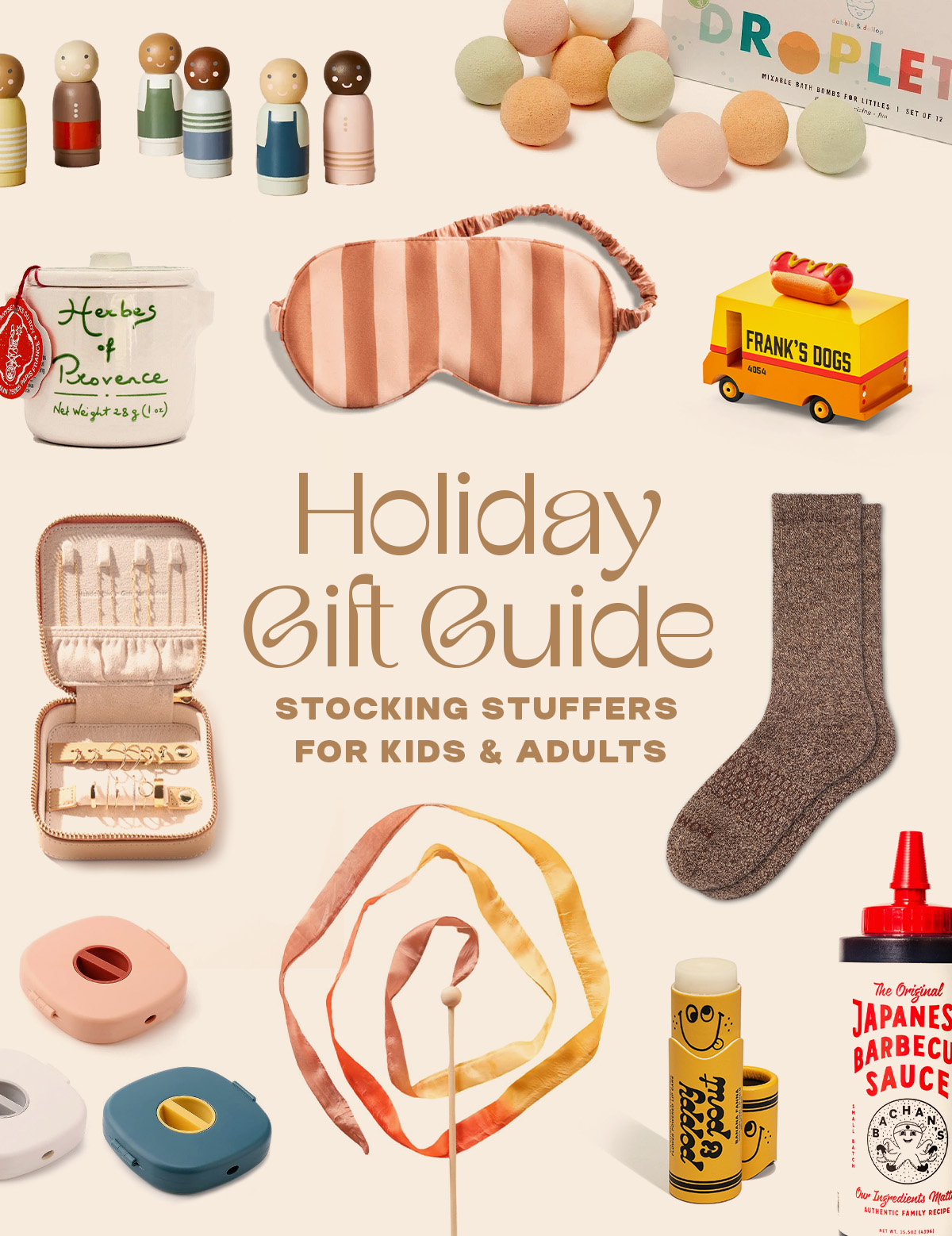The image is an advertisement for a Holiday Gift Guide featuring Stocking Stuffers for Kids and Adults, set against an off-white or cream-colored background. Centralized text in brown reads "Holiday Gift Guide, Stocking Stuffers for Kids and Adults," with various gift items meticulously arranged around it. 

In the top left corner are simple, minimalist figurines with cylindrical bodies and circular heads, showing basic facial features. To their right are pastel-colored bath bombs labeled "droplet." 

Below these, on the left side, is a white cookie jar with green text that says "Herbs of Provence." Adjacent to this jar is a pink and peach-colored sleeping mask featuring vertical lines. To the right of the mask is a toy van, orange and yellow in color, with a hot dog illustration on the top and labeled "Frank's Dogs."

Flanking the central Holiday Gift Guide text are additional items: a jewelry case on the left and a pair of brown socks on the right. 

At the very bottom of the image, on the left, are small plastic objects with a turnable part for fingers, likely a simple toy or gadget. To their right is a waving stick wrapped in cloth, followed by what looks like a lip balm, and on the far bottom right corner, a container of Japanese barbecue sauce.

These diverse and thoughtfully presented items showcase a range of fun and practical stocking stuffers suitable for both kids and adults.